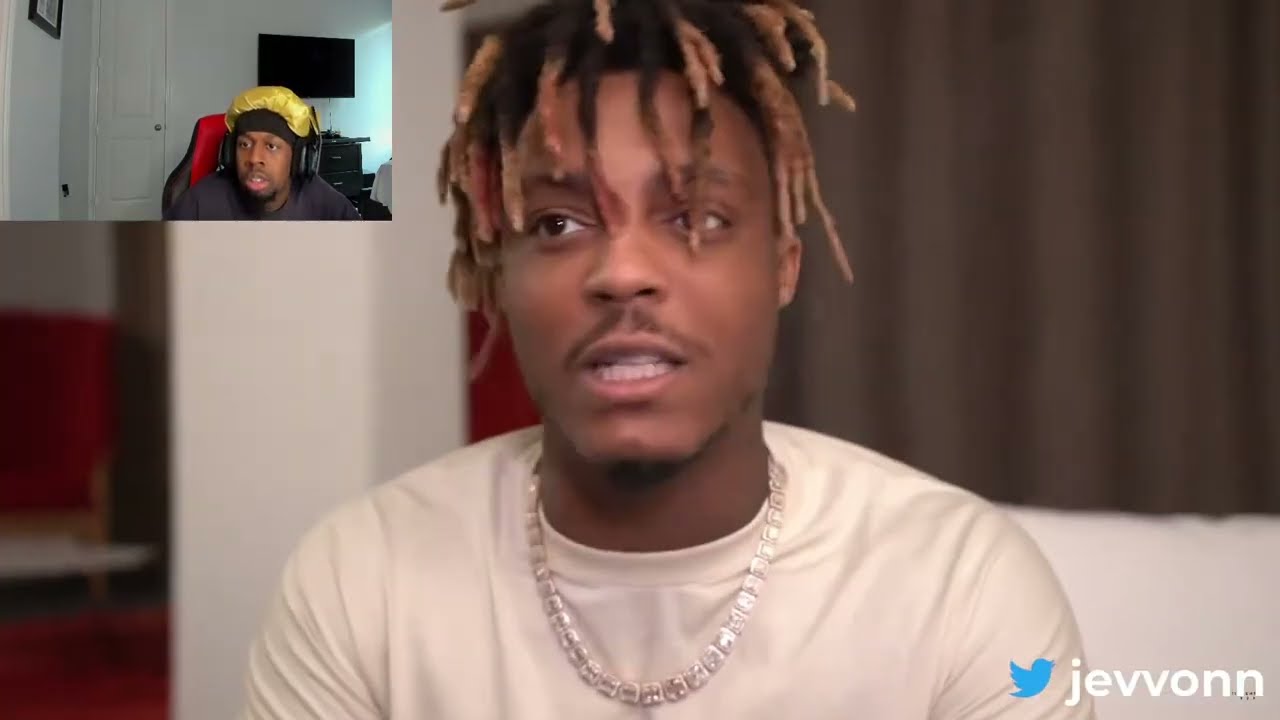This indoor, horizontally-oriented color photograph captures a young Black man in his twenties, wearing a silver necklace and a white t-shirt. His hair is styled in plaits with frosted ends, and he sports a scruffy black mustache and a slight beard. The setting appears to be a casual living space with a grey and dark brown curtain as the backdrop, partly covering a distant white wall, a door, a flat screen TV, and a framed image. Dominating the bottom right-hand corner is the old Twitter graphic and the text "J-E-V-V-O-N-N" in lowercase white letters.

Inset in the top left corner, a secondary image shows another African American man with a thin mustache and beard. He is wearing a black hat with a yellow brim and a headset, seated in a red chair. His mouth is open, indicating he is speaking. This inset suggests the main subject is engaged in a video call. The combined elements create a rich, social media-style photograph, capturing an informal moment of connection between the two men.